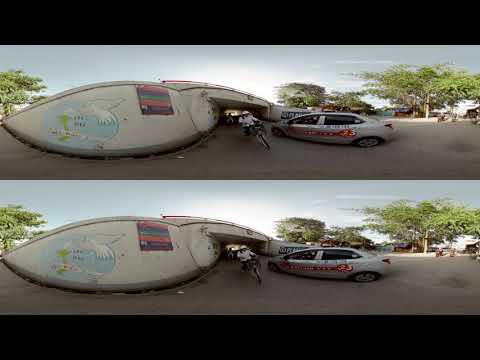The composite image features two identical, horizontally aligned photographs, one positioned above the other, each bordered by black bars at the top and bottom. Both images present a somewhat blurry and pixelated outdoor scene. Dominantly, the foreground showcases a bicyclist emerging from the shadowed passage of a curving, white stone tunnel or bridge. 

To the right of the bicyclist, a grayish-white sob car, bearing blurred advertisements or decals along its side, appears to be moving toward the tunnel. On the far-right side of the image, a stretch of paved road extends outward, interspersed with three tall, fully-leaved trees that stand vividly green. A fourth tree appears from the other side of the screen along with a long, cement wall curving parallel to the road, enveloping the scenery in a continuous sweep.

Clouds, a partial view of the sun, and a blue sky form the backdrop, adding light to the image and emphasizing its daytime setting. Numerous pixelation issues make finer details like the text on the vehicle and possible graffiti on the tunnel difficult to discern.